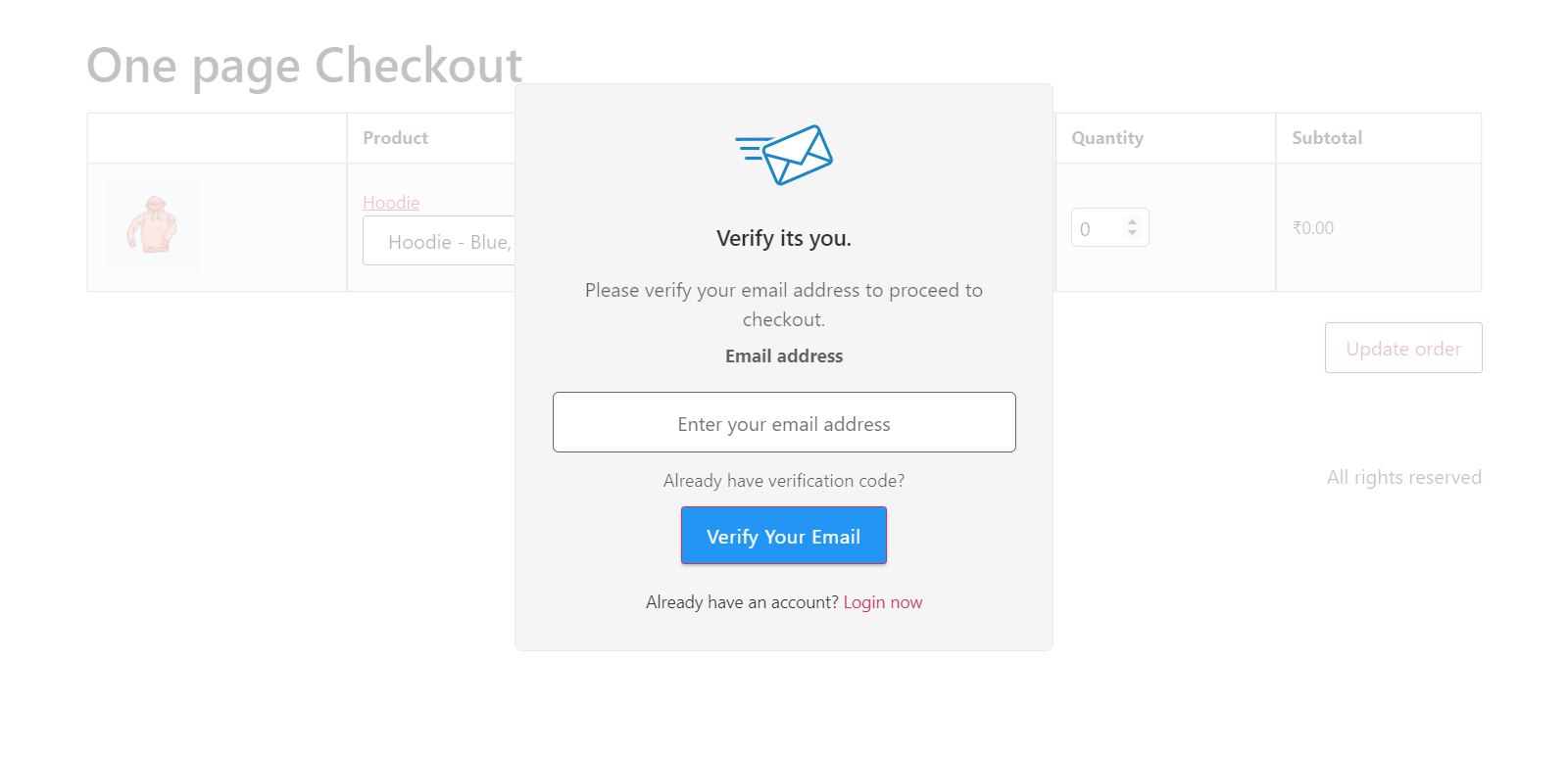The image depicts a checkout page with a "One Page Checkout" header located in the upper left corner. Central to the image is a gray pop-up window overlaying the checkout page. Prominently displayed within the pop-up is a stylized blue envelope icon, featuring three black lines emerging from its upper left side, giving the appearance of emanating communication.

At the top center of the pop-up, bold black text reads "Verify it’s you". Below this, in a lighter gray font, the instructions state, "Please verify your email address to proceed to checkout". Proceeding downward, the term "Email address" appears in black font, signifying the required field.

Directly beneath, a text input box is presented for users to enter their email addresses. Completing the form, a blue button labeled "Verify Your Email" is available for users to click and confirm their email address, thereby allowing them to proceed with the checkout process.